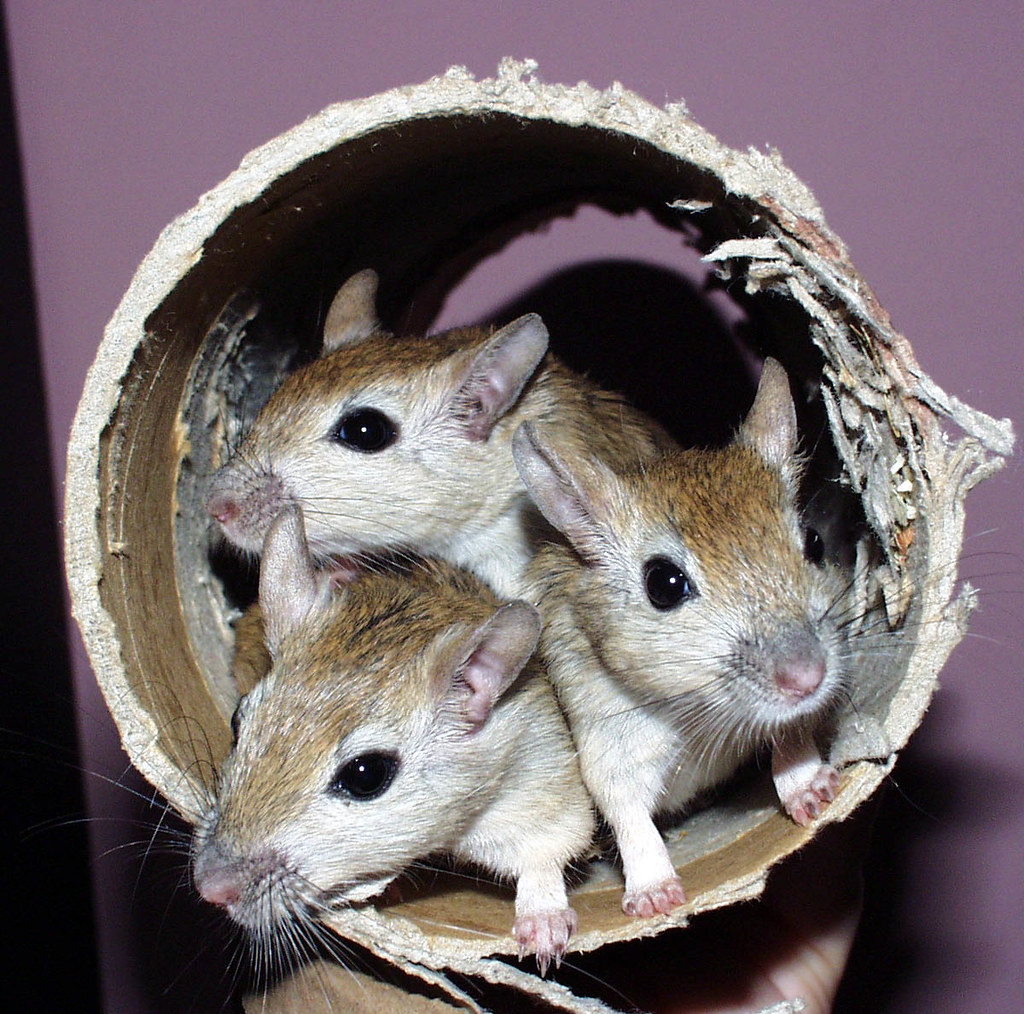This is a detailed color photograph capturing three young mice crowded together inside a ragged, chewed-up cardboard tube. Their bright black eyes, pink noses, and long whiskers stand out, with mostly brown fur accented by lighter coloring on their throats and chests. The mice, tightly packed at the bottom of the tube, display their little pink paws and claws. A hand, barely visible with just a fingertip showing, holds the tube. The background is a mauve or medium purple, adding a soft contrast to the scene.